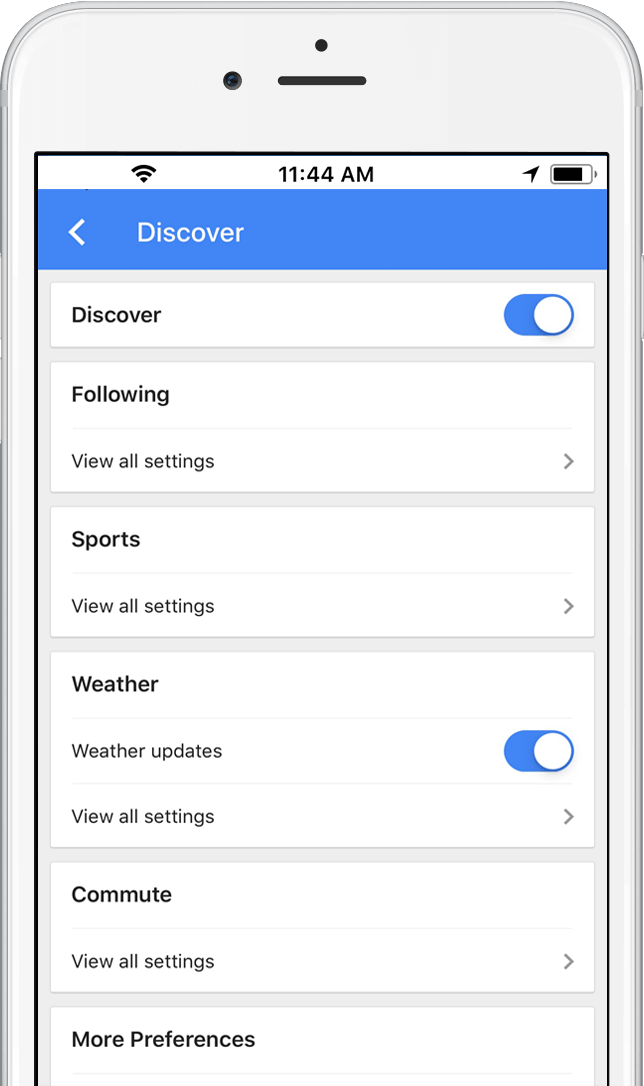The image showcases a white iPhone displaying an app interface, specifically the "Discover Settings" screen. The app, possibly an all-in-one assistant similar to Siri or Google Assistant, allows users to toggle various features on and off. At the top of the screen, the word "Discover" is prominently displayed, indicating a section within the app. Below it, there are multiple settings options such as "Sports," "Weather Updates," and "Commute," each with the ability to be turned on or off via blue toggles. The background is predominantly white, contrasting with black text and blue toggles. At the top left, there's a back button, and the status bar shows the iPhone's battery is nearly full, the location service is active, Wi-Fi is connected with a strong signal, and the current time is 11:44 AM.